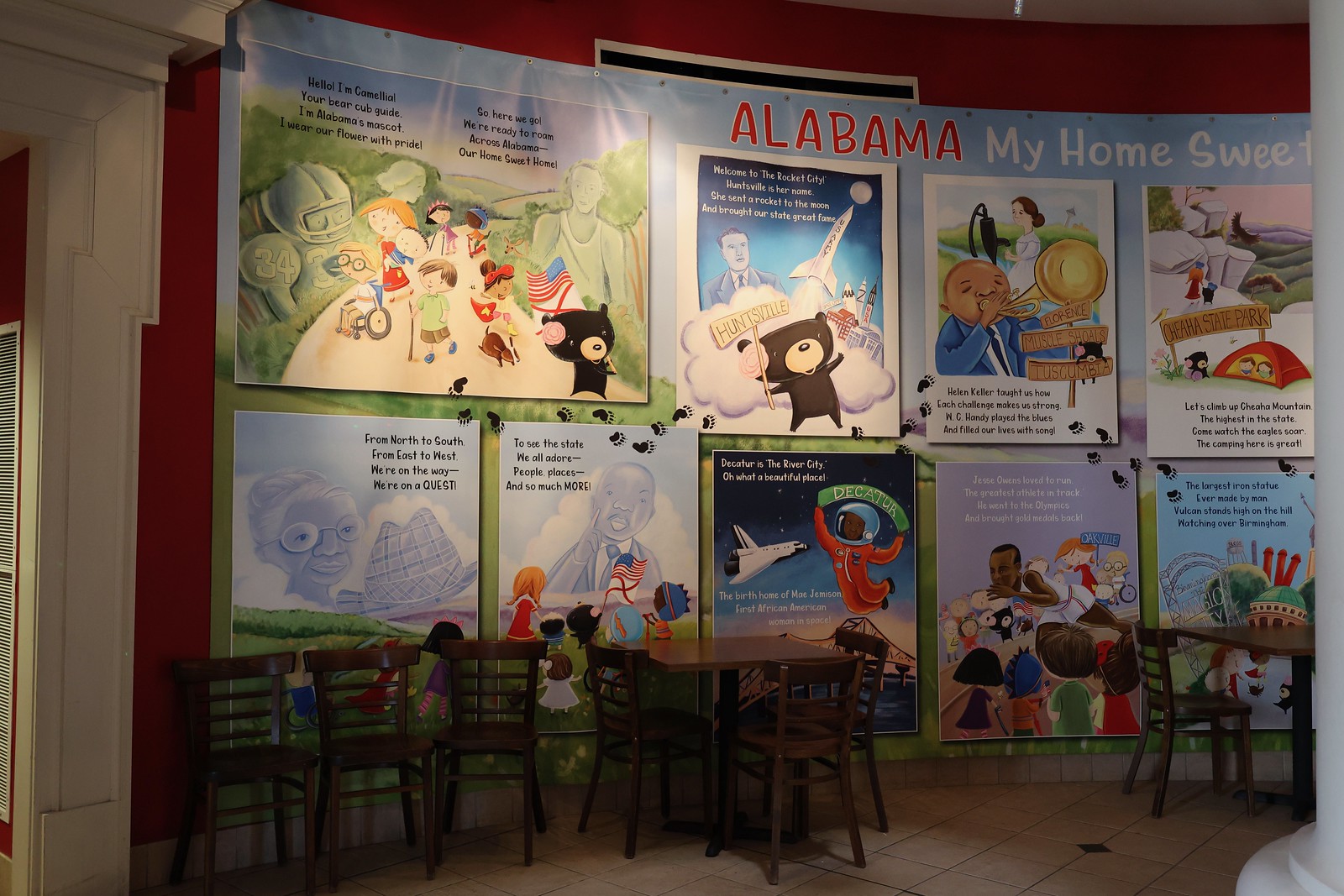The image depicts an indoor sitting area with a tile floor, featuring wooden tables and chairs lined up against a vibrant red, semi-circular wall. Prominently displayed at the top of the wall in bold, uppercase red letters is the partially cut-off text, "ALABAMA MY HOME SUITE." The wall is adorned with a series of large, colorful posters, which appear to be children's illustrations. These illustrations include images of an elderly woman, Martin Luther King Jr., a black bear holding a sign that says "Huntsville," and children running down a dirt trail. Other posters show scenes like a person playing a trumpet, a rocket, and a basketball player, all crafted in a cartoonish style. The room also includes a white-bordered entranceway on the left side of the red wall, enhancing the lively and playful ambiance with a mixture of historical and whimsical imagery.